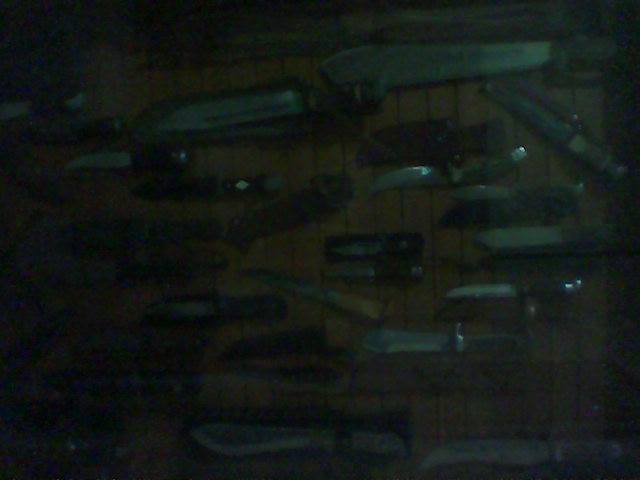This photograph is an extremely low-quality, underexposed color image depicting what appears to be an assortment of knives and metal tools scattered on a wooden surface. The image is very dark and blurry, making it difficult to discern precise details. However, numerous items seem to be knives with sharp, pointed stainless steel or silver blades, some longer than others. The blades catch minimal light, revealing faint reflections. Most of them are oriented towards the left side of the frame while lying on a surface with visible vertical wooden panels. Among the various items, one knife in the middle stands out with a lighter, almost light brown handle. Additionally, some knives seem to be in sheaths, indicative of hunting knives rather than kitchen knives. Tiny brown squares are also attached to the wooden backdrop, possibly serving some display or mounting function. The photograph appears to have been taken in a dimly lit, enclosed space, potentially a dark closet or shed, without the use of a flash.